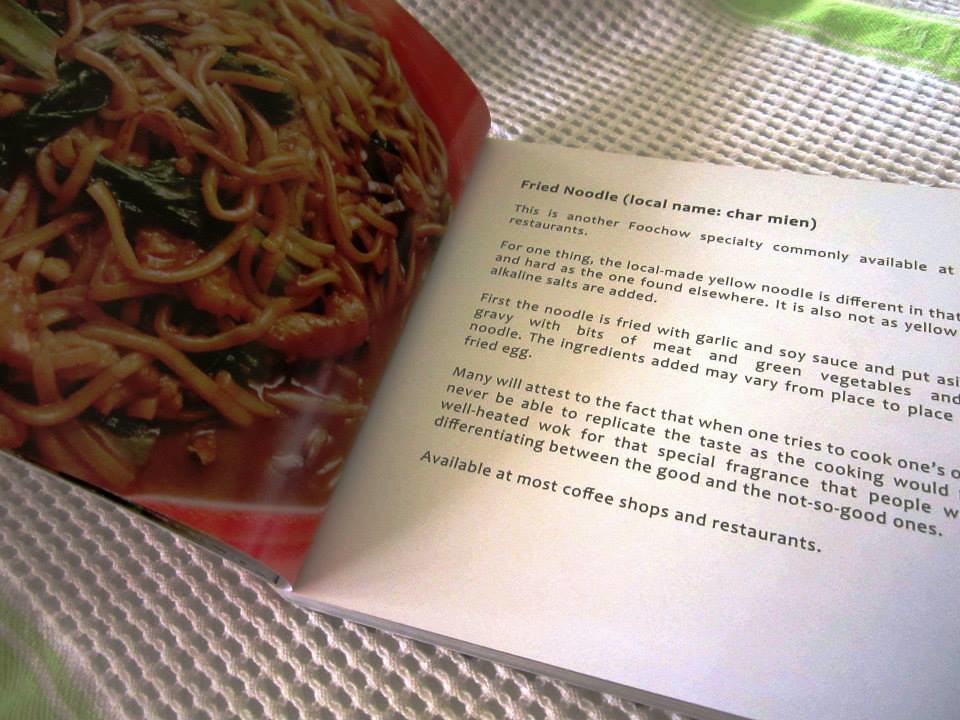The image is an overhead photograph of an open horizontal cookbook, showcasing a recipe for fried noodles called "Char Mien". The left-hand side of the book displays a vibrant photograph of the dish in a red bowl, featuring yellow noodles garnished with pieces of meat and green leafy vegetables. The noodles appear browned from frying and are covered in a savory sauce. The right-hand page, set against a white background with black text, describes Char Mien as a local Fu Chao specialty commonly available at restaurants, distinguishing itself with its locally-made yellow noodles that are harder and more vibrant, due to the addition of alkaline salts. The recipe explains that the noodles are first fried with garlic and soy sauce before being combined with gravy, bits of meat, green vegetables, and occasionally a fried egg. The text emphasizes that the unique flavor, which many find difficult to replicate at home, is achieved by cooking the noodles in a well-heated wok, a technique that imparts a special fragrance. Although some of the text on the right page is cut off in the photograph, it concludes by stating that Char Mien is widely available at most coffee shops and restaurants. The background of the image includes a white tablecloth with green trim on the corners.